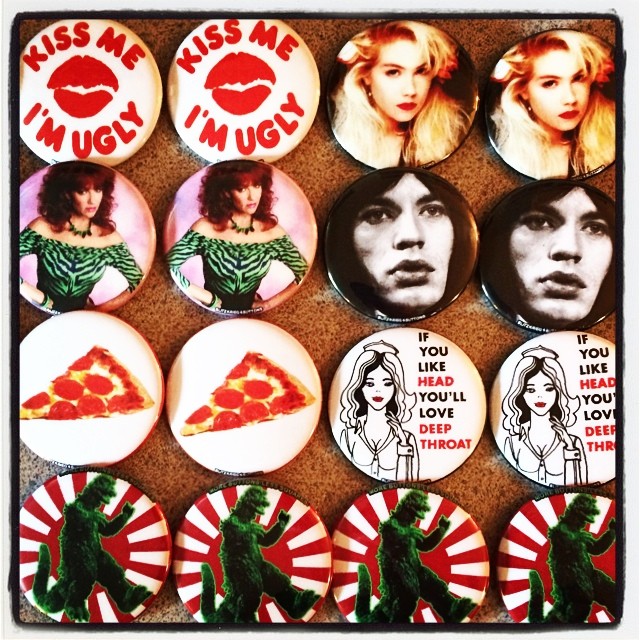This image features a corkboard displaying a 4x4 grid of 16 circular buttons, resembling those used for campaigns or jean jackets. Each button is pinned in pairs, and one design appears four times. Starting from the top-left: the first pair of buttons reads "Kiss Me" with lips illustrated between the phrases, followed below by "I'm Ugly." To the right, there's a close-up of a glamorous woman with blonde hair and red lipstick.

Moving to the second row, the left button displays a brunette woman in an 80s-style outfit, specifically a zebra print top. Next to her is a close-up black-and-white image, of a person with dark hair, resembling Mick Jagger. 

The third row begins with a slice of pepperoni pizza on the left, followed by two identical buttons featuring a nurse with a provocative caption: "If you like head, you'll love deep throat."

Finally, the bottom row consists of four identical buttons featuring a classic Godzilla image set against a backdrop resembling a Japanese rising sun or possibly a poker chip with red and white stripes.